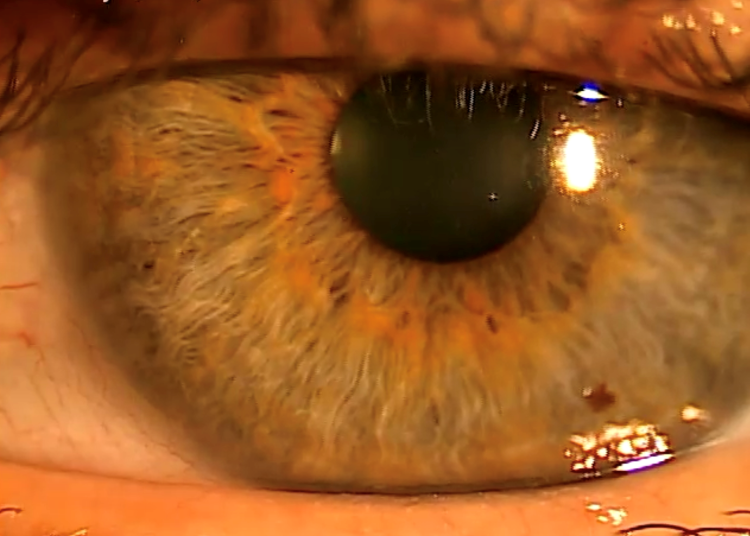This photograph, captured in landscape orientation, is an extreme close-up or macro shot of an eye. The eye appears hazel, yet it exhibits a mesmerizing blend of green, yellow, gold, brown, and even hints of blue, giving it a dynamic, almost surreal appearance. The glossy nature of the eye accentuates its wetness, with visible light reflections creating splotches on the iris and a stark highlight on the right side. The upper eyelid is partially closed, causing the eye to squint slightly, with the upper eyelashes dipping down into the frame and a few lower eyelashes also visible. The skin of the eyelids shows intricate details with off-white and brown speckles. The whites of the eye reveal subtle veins, enhancing the lifelike quality of the image. The overall effect is striking and somewhat eerie, with the eye filling the entire frame and no parts of the surrounding face visible.